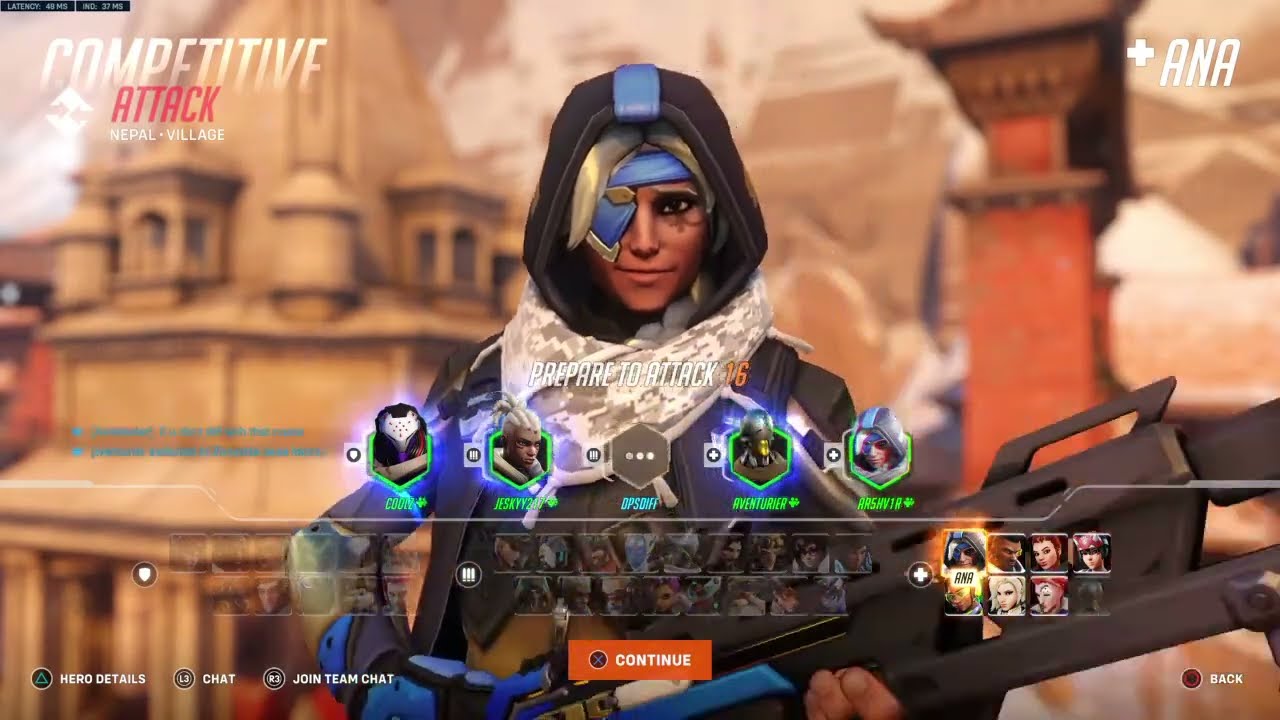This is a detailed screenshot from a video game called "Competitive Attack," likely taken from a character selection screen. The image features a female soldier as the primary character, who is heavily equipped and prepared for combat. She is dressed in multiple layers of blue and black clothing, possibly armor. Notably, she wears a beige and brown camo-patterned scarf around her neck, and on her head rests a gray hood with a distinctive blue stripe running down the center. Adding to her unique appearance, she has a blue headband with an eye patch covering her left eye, leaving her right eye visible. Her hair is a striking whitish-blonde.

The soldier holds a large, futuristic rifle with both hands—the right hand gripping the back and the left hand supporting it underneath. She stands against a blurred backdrop featuring brown, orange, and white stone buildings, giving the scene a futuristic urban vibe. 

In the upper left corner of the screen, the words "Competitive Attack" appear in white, followed by "Nepal Village" in red. The top right corner shows a plus symbol followed by "ANA" in white. The bottom of the screen is populated with various interface elements: a "Continue" button in the center, "Hero Details," "Chat," "Join Team Chat" on the lower left, and a "Back" button on the lower right. Additionally, small character avatars are scattered across the bottom, indicative of other playable characters and the player's chosen lineup. The text "prepare to attack" is also displayed, with a countdown timer, indicating an imminent game start.